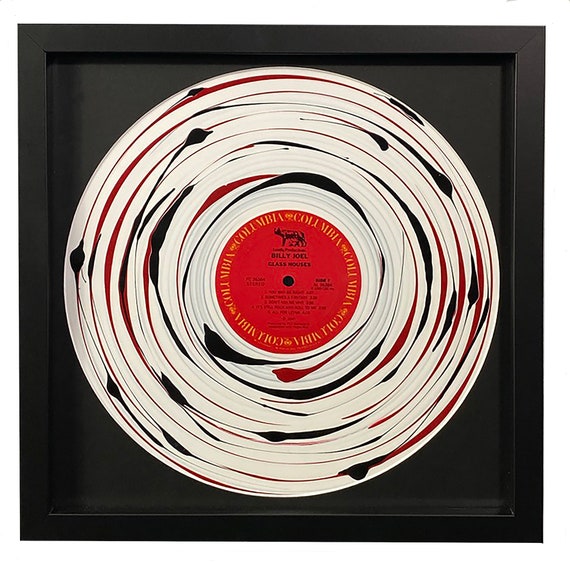The image depicts a framed vinyl record album, specifically Billy Joel's "Glass Houses" under the Columbia label. The record is encased in a black frame, with the frame's outer edge protruding slightly more than the record itself, creating a recessed appearance. The vinyl appears to have been creatively altered; it has a white base color with dynamic streaks and splotches of red and black paint applied in a circular and somewhat irregular pattern. The central part of the record features the Columbia label, with "Billy Joel" written in prominent black text surrounded by a red circular area. Additionally, there is a depiction of a rhinoceros near the top center of the red circle. Despite the alterations, which seem to aim for an artistic effect, the result contrasts sharply with the original red and yellow colors of the Columbia label, giving the record a somewhat disjointed appearance.